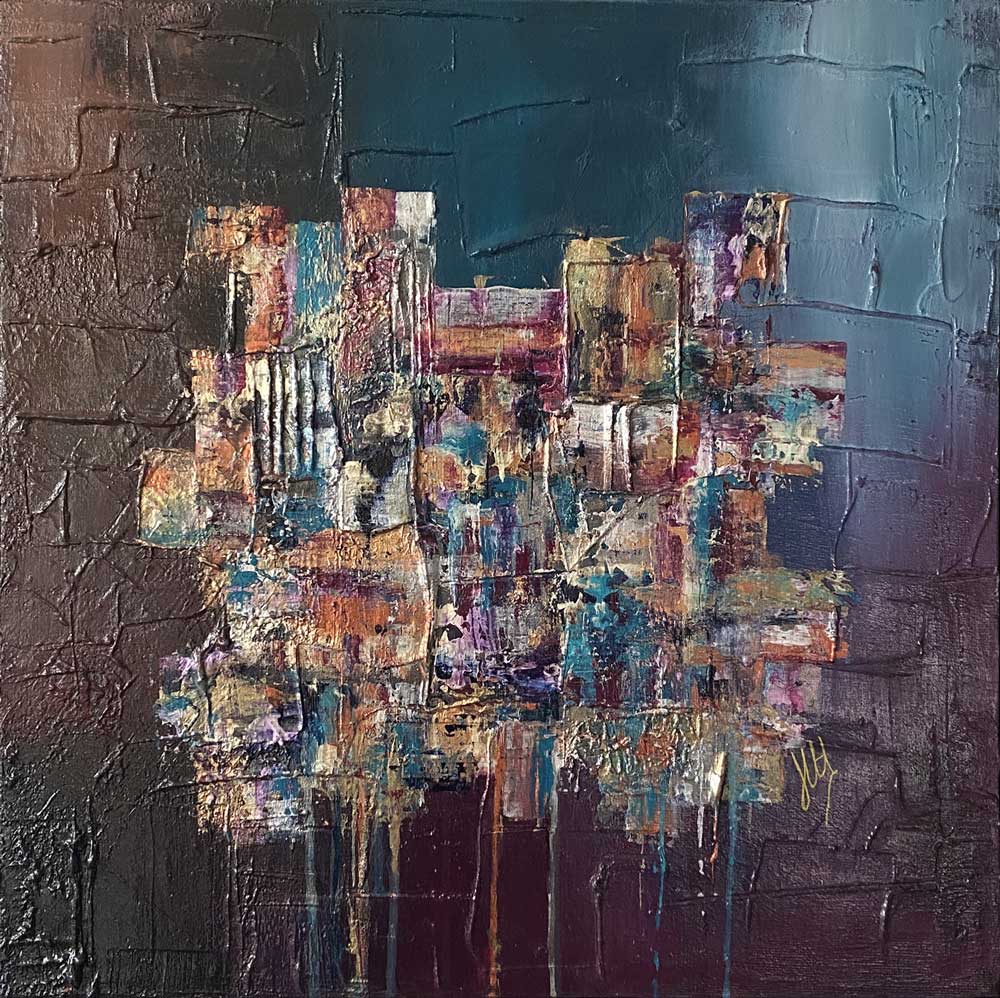The image depicts an abstract painting on a large stone wall, possibly captured outdoors. The painting is textured and appears to be done on canvas. On the upper left side, the dominant color is brown, while the top right transitions from blue to a deep plum color towards the bottom. The lower left corner features a deep green hue. The central portion of the painting is an eclectic explosion of colors—including orange, yellow, and blue—applied seemingly with a sponge, creating a mosaic effect with strokes in various directions. This central area has an embossing effect, making it stand out against the multicolored background. The colors appear to bleed and drip downwards, especially noticeable at the bottom of the image. The painting lacks any specific structure or pattern, embodying a purely abstract form. Near the bottom right corner, the artist’s signature is visible in yellow.